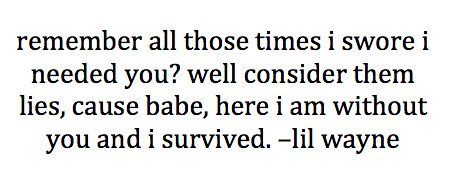The image features a white background with four lines of black text in a simple font. All the text is in small caps and there is consistent spacing between each word. The quote reads: "remember all those times i swore i needed you? well, consider them lies, cuz babe, here i am without you and i survived." A dash follows this quote, attributing it to "lil wayne." The text is notably uncapitalized, including the pronoun "i" and the name "lil wayne." There is no other content in the image, making the focus solely on the quote.